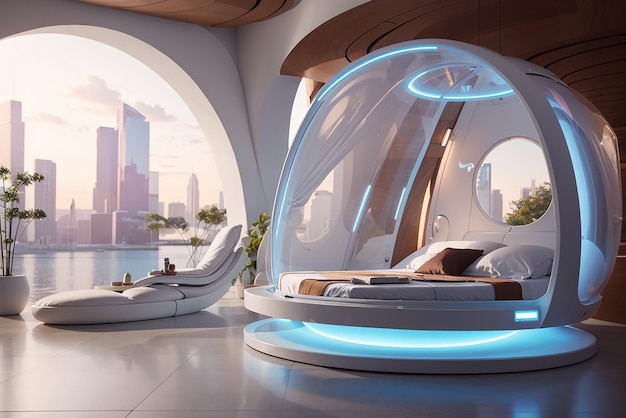The image depicts a highly futuristic and modern bedroom with a stunning view of a city skyline across a body of water, possibly a lake or ocean. A large, arched window that spans nearly the entire wall offers this panoramic view. Central to the room is a unique sleep pod, featuring a bed encased within a large, dome-like structure illuminated by neon turquoise and blue LED lights. The pod appears elevated and mechanized, with white panels and a small circular viewport at its rear. Inside, the pod contains a standard mattress and pillows, giving it a capsule-like appearance. On one side of the room, a sleek lounge chair accompanied by a small table and a potted plant provides additional comfort. The overall design of the room is posh, slick, and exudes a sense of luxury and modernity.